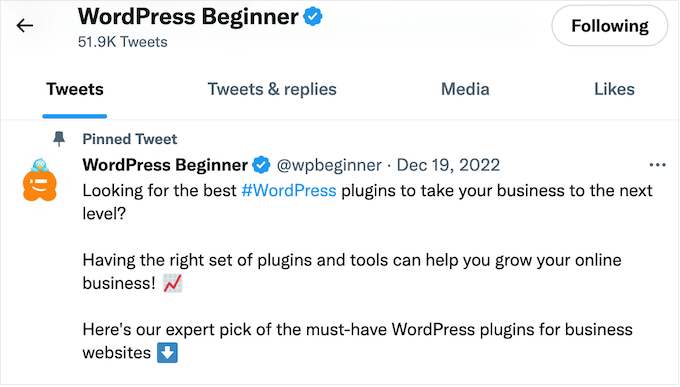The image depicts a Twitter interface, viewable on both computers and smart devices, framed by a thin gray border that contrasts slightly with the white background of the device. 

In the upper-left corner, there is a black back arrow. Next to the arrow, "WordPress Beginner" appears in bold black font, accompanied by a blue circle containing a white checkmark. Below this, in a less bold font, is text indicating "51.9K Tweets." In the upper-right corner, there is a follow button.

Below this section, various tab options are displayed, with "Tweets" selected, appearing bold and underlined in blue. Additional tabs for "Tweets & Replies," "Media," and "Likes" are present but not selected. A thin gray line separates these tabs from the main content.

The main content starts with a pinned tweet indicator, marked by an orange pushpin icon. The tweet itself is from "WordPress Beginner," with the same blue circle and checkmark. The username "@wpbeginner" and the date "December 19, 2022," are also listed. The tweet promotes essential WordPress plugins, stating: "Looking for the best #WordPress plugins to take your business to the next level? Having the right set of plugins and tools can help grow your online business. Here’s our expert pick of the must-have WordPress plugins for business websites." There is an icon at the end of the tweet.

Below the tweet, there is a blue box with a white downward-pointing arrow.